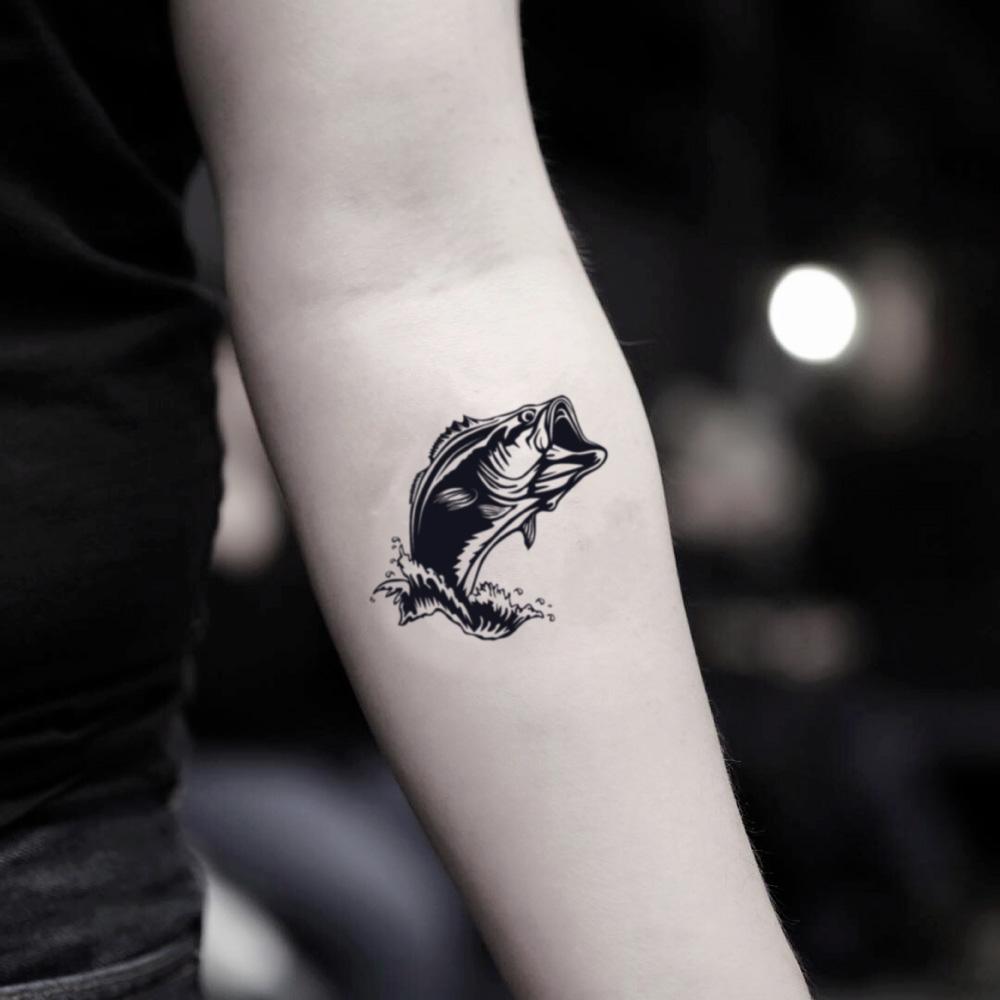This photograph features a close-up of a person's left arm, which is illuminated possibly by a camera flash. The individual is wearing a black shirt, and dark jeans, which are barely visible on the left edge of the image. The background is heavily blurred and dark, suggesting the photo might have been taken at night. The arm, depicted from the mid-bicep down to just above the wrist, showcases a black-and-white tattoo of a largemouth bass leaping out of water, situated just below the elbow. The fish's mouth is open, with an expressive gaze and spiked fins along its back. Detailed in a simple yet bold illustration style, the fish bears a resemblance to the Bass Pro Shop logo. A hint of a white border suggests that the tattoo might be photoshopped onto the arm, as the blend is not entirely smooth. Additionally, a single circular bright light appears just above the center line on the right-hand side of the image.